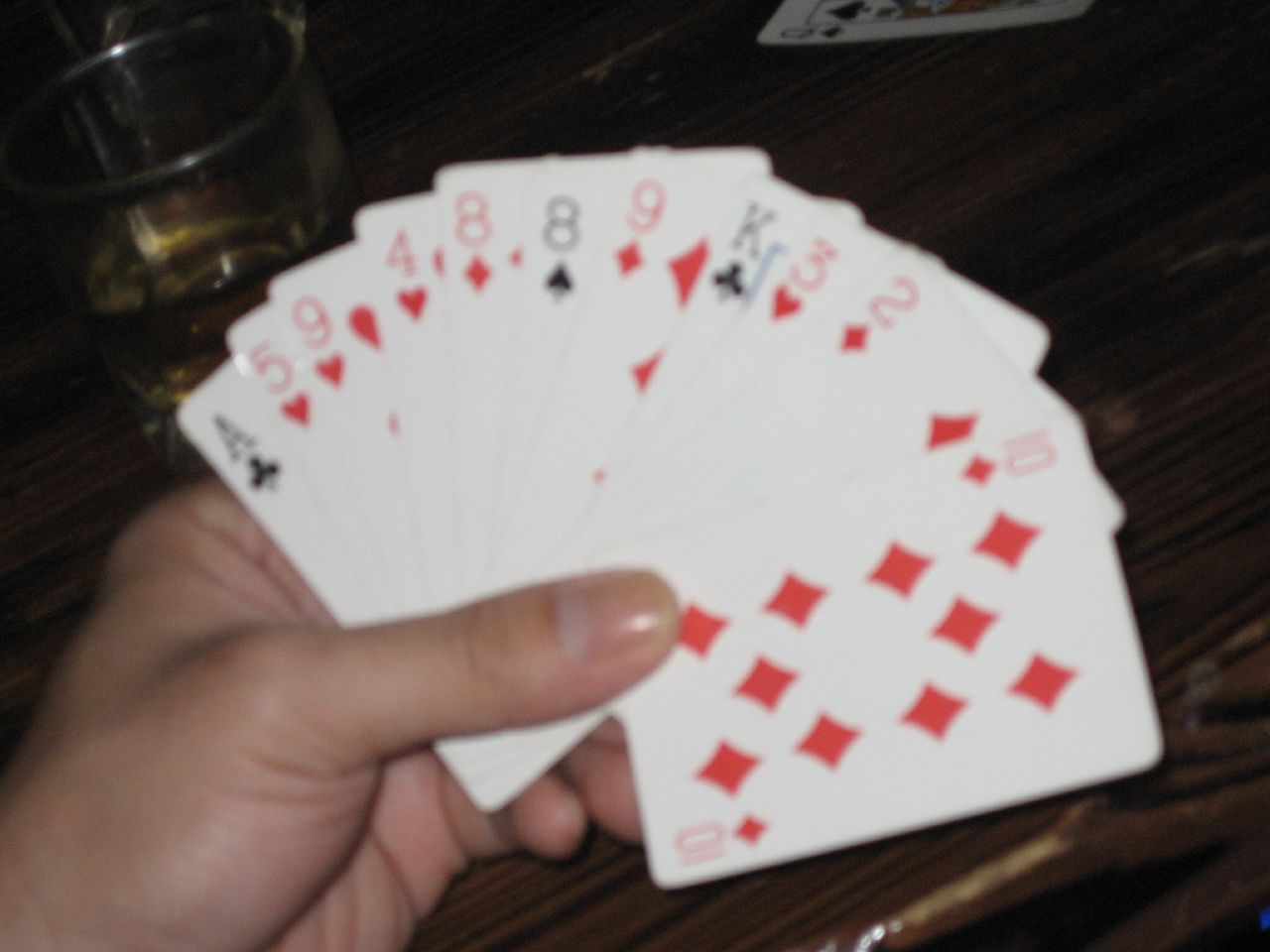In a dimly lit setting, a photograph captures the left hand of an individual holding a fan of playing cards. The cards are meticulously spread out in a cascading sequence, creating the impression of either a mid-performance magic trick or a moment within a captivating card game. The fan of cards prominently displays the ten of diamonds at the top, followed by the two of diamonds, three of hearts, king of clubs, nine of diamonds, eight of clubs, eight of diamonds, four of hearts, nine of hearts, five of hearts, and the ace of clubs. In the background, the dark ambiance is softened by the presence of a drink placed to the left on the table, hinting at a relaxed, social atmosphere. This setup suggests that the person is seated comfortably at a table, carefully arranging their cards in front of them, poised either for a reveal or simply for the camera's capture.